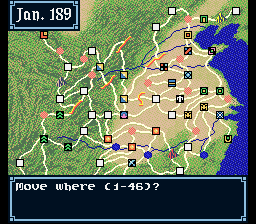This screenshot captures a vintage computer game featuring a detailed map interface. The map is composed of white outlined pathways, resembling roadways, interspersed with small squares of various colors and designs. Each square seems to signify different elements or locations within the game. In the top left corner, there is a rectangular black box with a white border that reads "Jan. 189." At the bottom of the screen, spanning from left to right, another black box displays the prompt "Move to where, 1-46." The entire image exudes a nostalgic feel, characteristic of early computer games, with its simplistic yet intricate design elements.